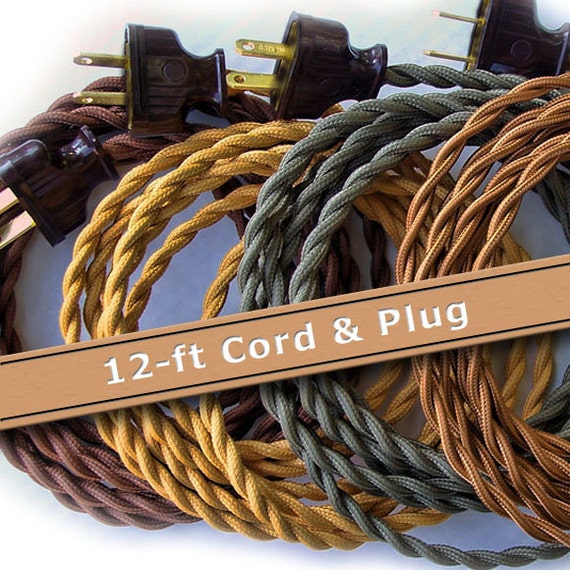The image displays a square photograph, approximately four inches by four inches, showcasing four electrical cords and their corresponding plugs. At the top of the image, above a lime green background, four black plugs with bronze prongs are neatly aligned. Below the plugs, the cords themselves are coiled into tight spirals of different colors and are positioned against a blue background.

Starting from the right and moving clockwise, the first cord is a light brown, leather-like material with black stitching, prominently featuring a white stamp that reads "12-FT Cord and Plug." The second cord is a grayish-blue shade, followed by a golden-yellow cord, and finally, a cord in a reddish-purple hue. Each cord is made from a braided nylon material, wrapped in distinct, visually appealing loops.

In the center of the image, a banner clearly states "12 foot cord and plug," emphasizing the length and dual functionality of the items displayed. The overall composition is neat and detailed, highlighting both the aesthetic variety and consistency in design of the cords and their plugs.